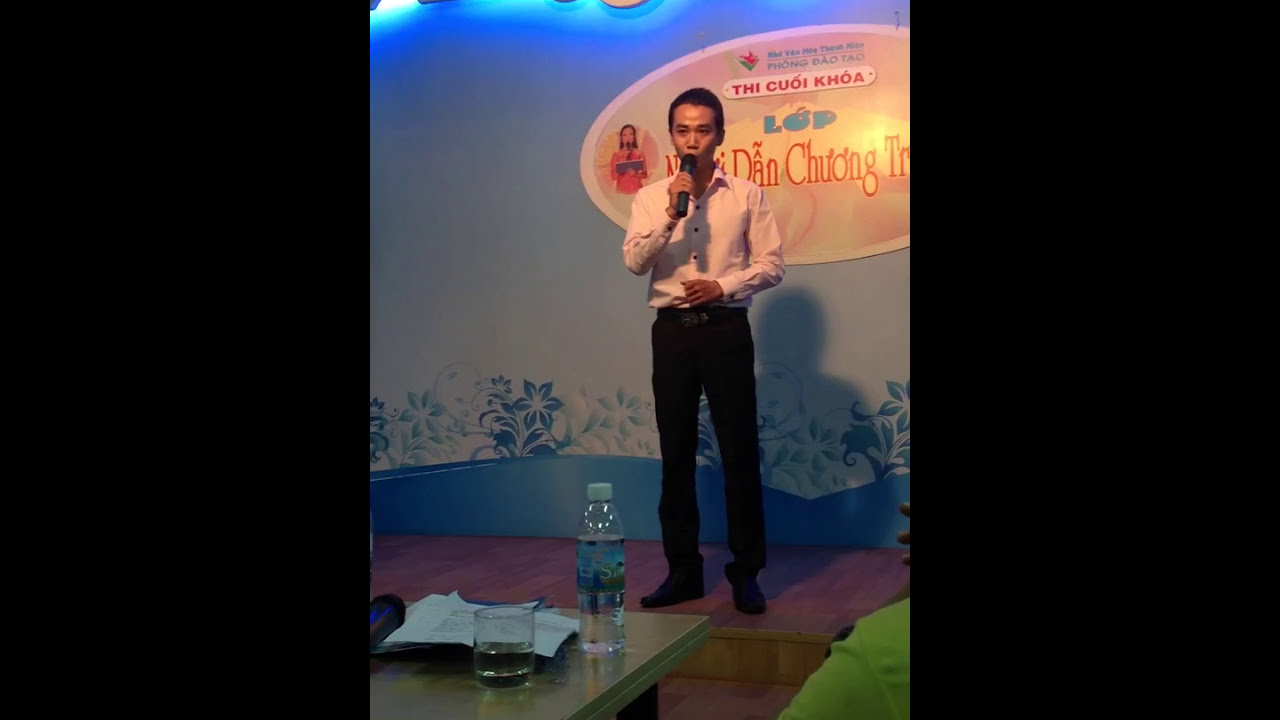A young, slender Asian man in black dress shoes, black pants, and a salmon-colored button-down shirt stands on a small wooden laminate stage. He holds a black microphone to his mouth, appearing to speak or sing. The backdrop features varying shades of blue and includes a sizable, orange sign with undecipherable text in a foreign language. On a glass-topped table in front of him, there are a bottled water, a glass, and some papers, suggesting he is delivering a presentation. The stage setting is indoors, with a photograph or still shot capturing the scene. In the bottom corners of the image, part of another person’s shoulder and the table are visible.